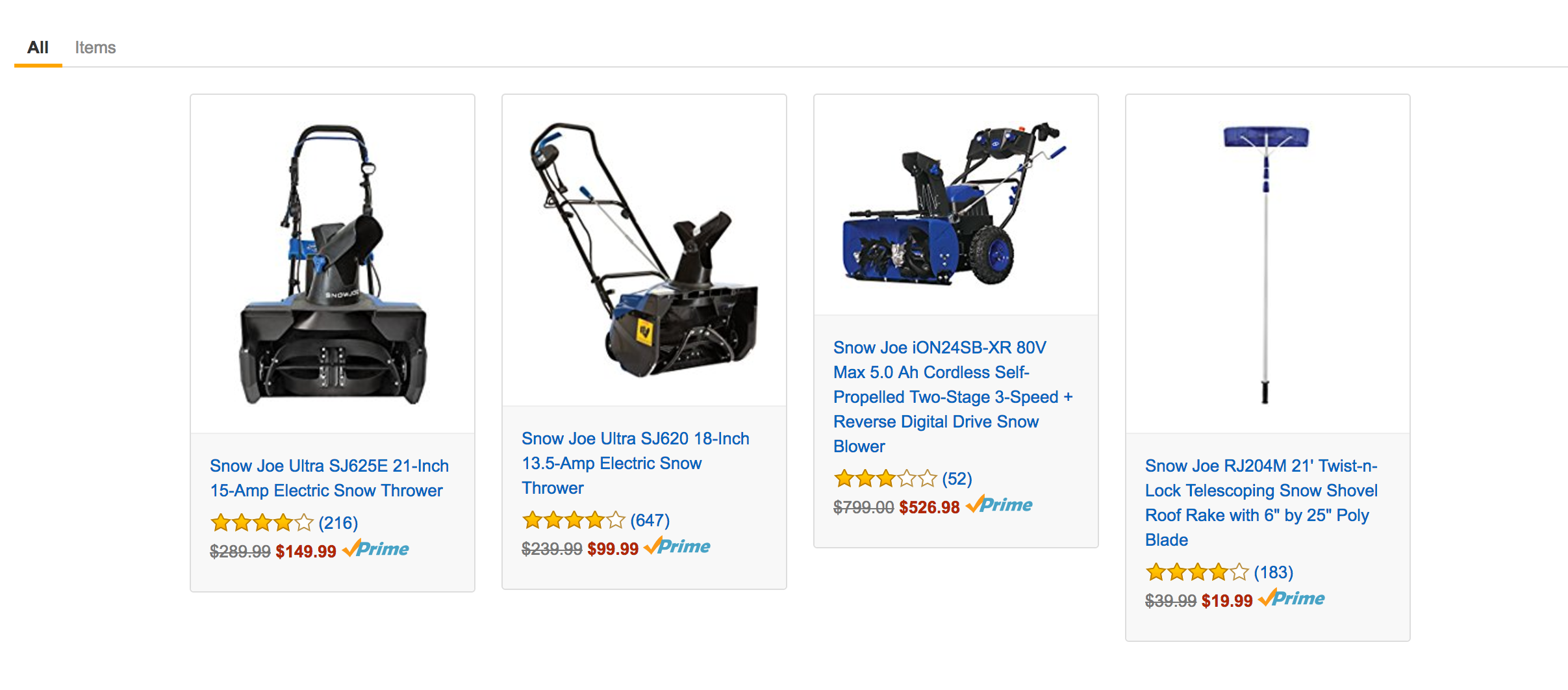Here is a detailed descriptive caption based on the cleaned-up information:

---

In the top-left corner of the image, there is text in yellow with grey underlining that reads "Items." The image prominently features three snow thrower products.

1. The first product is labeled with blue text, "SnowDrill Ultra SJ625E, 21-inch, 15 Amp Electric Snow Thrower." It has a rating of 4 gold stars, with one star hollow, and 216 reviews. The price for this product is marked as $289. However, there is no discount indicated.

2. The second product, written in red text, is the "SnowDrill Ultra SJ620, 18-inch, 13.5 Amp Electric Snow Thrower." Its listed price is $149.99.

3. The third product is described as "SnowDrill Ion 24SB XNR IDV, Max 5H, Cordless Hull Propeller, 2-Stage, 3-Speed Reverse Digital Dry Snow Blower." It has a rating of 3 gold stars, with two stars hollow, and 52 reviews. The price for this model is $526.99.

Off to the side, there is a mention of "SnowDrill RJ204M21, 2S10 Log, Telescopic Snow Thrower," featuring a 6 inch by 25 inch poly blade.

---